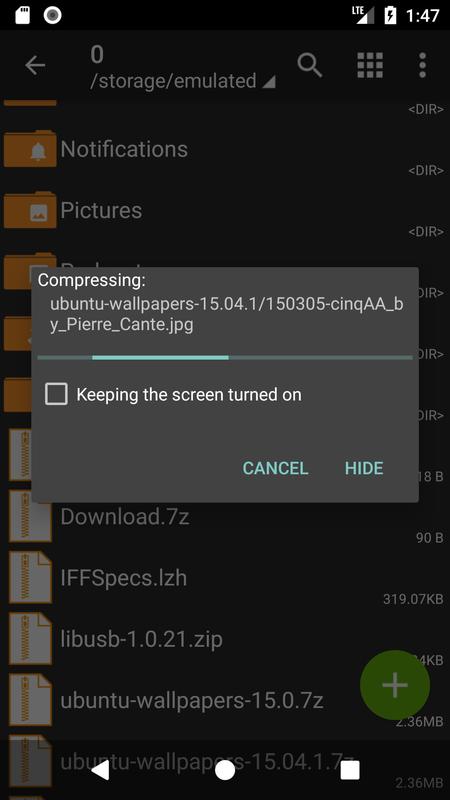The image depicts a high-resolution screenshot taken from a smartphone screen, focusing on a file compression task. The backdrop of the screen is solid black, providing a stark contrast that enhances visibility of the primary elements. Over this black background, a dark gray pop-up notification emerges, central to the image. 

The notification clearly indicates the ongoing process by displaying the text: "Compressing Ubuntu-Wallpapers-15.04.1/150305-SyncA_by_pierre_cante.jpg." This text elucidates that a specific file named "150305-SyncA_by_pierre_cante.jpg" from a directory labeled "Ubuntu-Wallpapers-15.04.1" is undergoing compression.

Within the notification, there are several interactive elements for user engagement. First, there is a checkbox option labeled "Keep screen on," allowing users to maintain the display's activity throughout the compression process. Below this, two actionable buttons are positioned: a "Cancel" button for terminating the process and a "Hide" button that allows the user to continue working without disruption while the compression occurs in the background.

In the less dominant section of the screen, behind the gray pop-up, the interface reveals the file directory structure of the smartphone. The specified directory path here is "/storage/emulated/," indicating local storage access. Within this directory, visible folders are labeled "Notifications" and "Pictures," suggesting an organized file management system.

Overall, the screenshot offers a meticulous view of the file compression interface on a smartphone, emphasizing the detailed text components, user-interactable options, and the underlying directory structure for an encompassing understanding of the scenario.